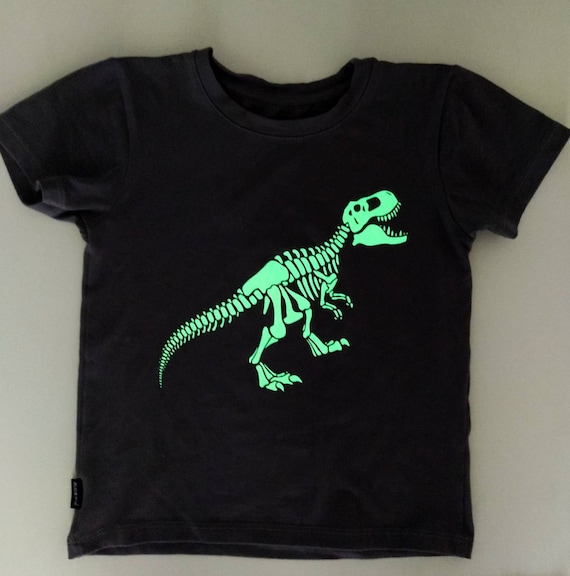This image depicts a black child-sized T-shirt with short sleeves, laid out flat on a beige table. The T-shirt features a striking neon green Tyrannosaurus Rex skeleton prominently displayed on the front. The T. Rex, depicted mid-walk with an open mouth, reveals detailed bones including eye sockets, teeth, vertebrae, bony legs, and feet. The skeleton appears almost luminous, possibly glow-in-the-dark, enhancing its vibrant presence against the black fabric. The T-shirt also has a scooped neck and includes a small tag on the bottom left seam. The overall presentation of the T-shirt suggests it might be intended for a product listing or a similar showcase, underscoring its appeal as a playful and eye-catching piece of children's clothing.